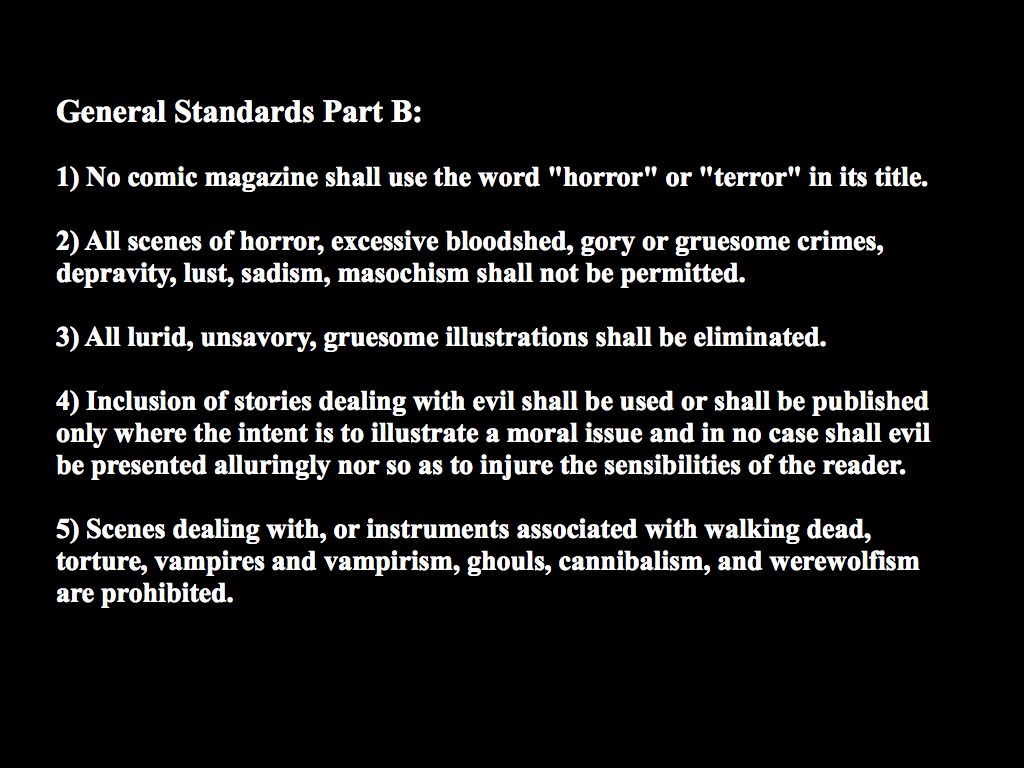The image features a solid black background with white text that reads "General Standards Part B" at the top. Below this heading, there are five numbered statements, each describing specific prohibitions for comic magazines. 

1. No comic magazine shall use the word horror or terror in its title.
2. All scenes of horror, excessive bloodshed, gory or gruesome crimes, depravity, lust, sadism, and masochism shall not be permitted.
3. All lurid, unsavory, and gruesome illustrations shall be eliminated.
4. Inclusions of stories dealing with evil shall be published only where the intent is to illustrate a moral issue, and in no case shall evil be presented alluringly, nor in a way that injures the sensibilities of the reader.
5. Scenes dealing with or instruments associated with the walking dead, torture, vampires and vampirism, ghouls, cannibalism, and werewolfism are prohibited.

The text is arranged neatly from top to bottom against the plain black background, making the prohibitions clear and stark.